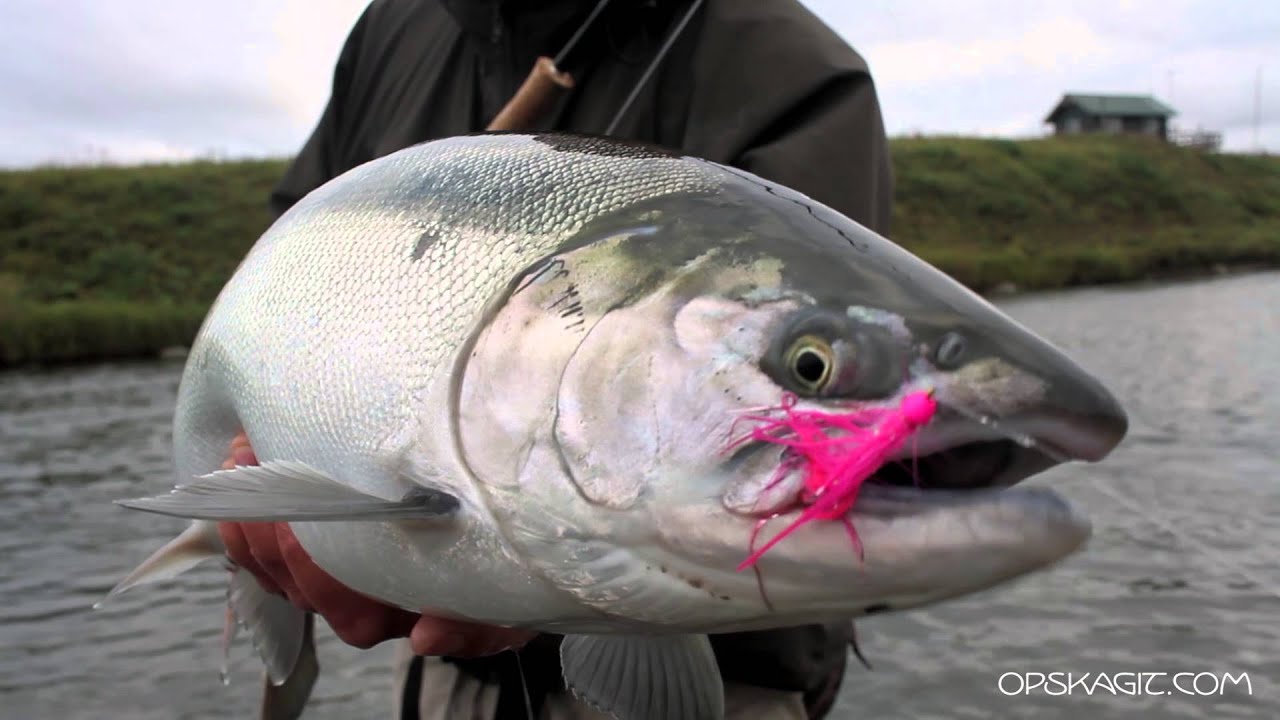In a close-up photograph from Opskagic.com, a man is proudly holding a large fish with a bright pink lure still embedded in its mouth, clearly connected to a fishing line. The fish, notable for its white belly and green-tinted top, almost matches the size of the man's torso, and is held horizontally with both hands. The man, dressed in a gray coat, is either standing in a river or right at its bank, surrounded by water that is not too deep. His face is out of frame, revealing only his hands, part of his upper body up to the shoulders, and a bit of his midsection. In the background, a grassy, sloped levee can be seen alongside a small green building in the distance. The overcast sky, filled with heavy clouds, casts a muted tone over the scene, hinting at a cloudy day.